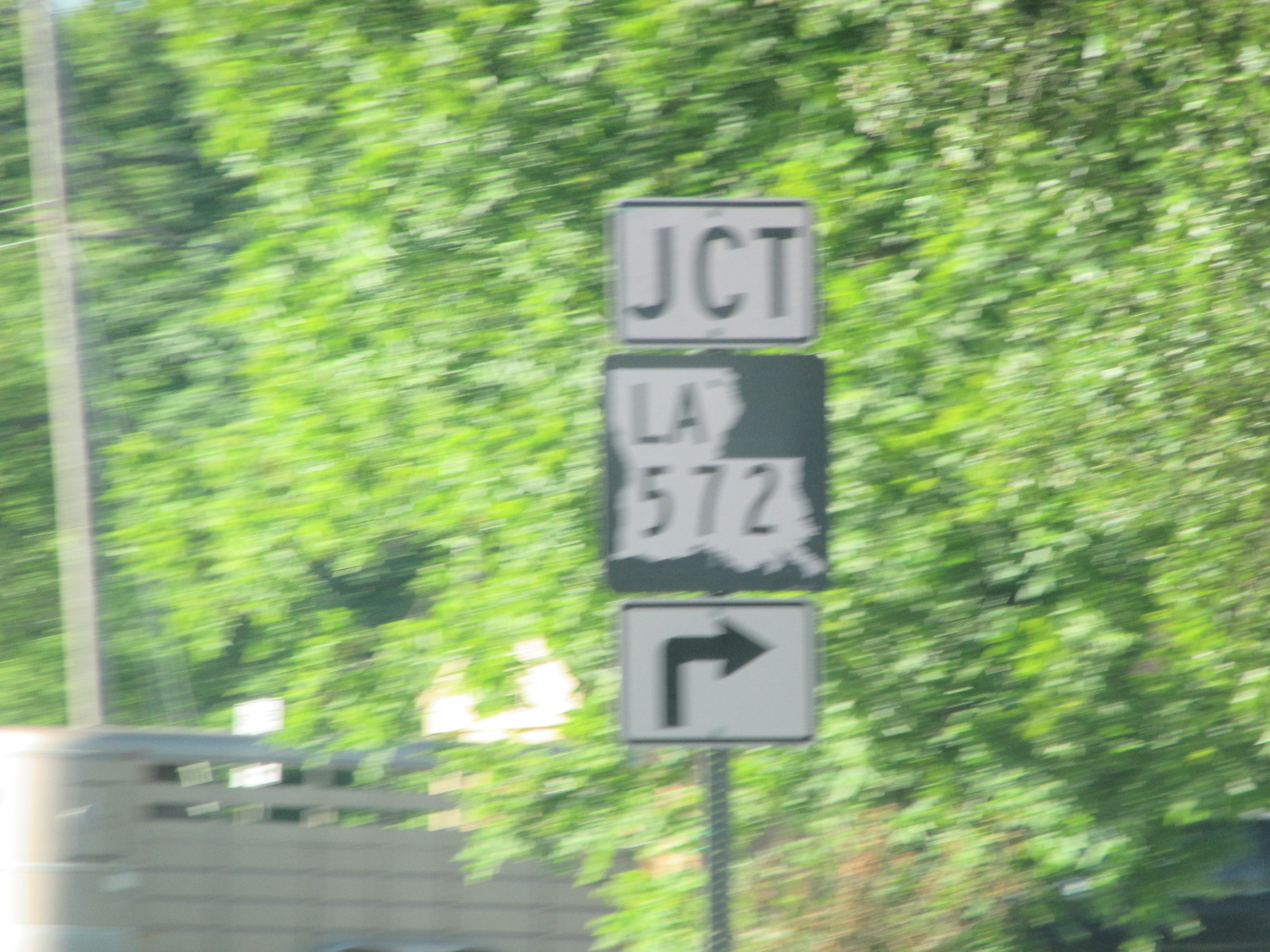This extremely blurry color photograph, seemingly taken from a moving car, captures a roadway scene dominated by greenery. The background is filled with a dense mesh of green leaves from trees. Positioned behind a wall or barrier at the edge of the image is a tall metal pole, partially cut off by the photograph's top edge. In front of the trees stands a shorter metal pole, which serves as the central focus of the image, adorned with multiple road signs stacked vertically. The topmost sign is a white rectangular plate bearing the letters "JCT" in large black font. Below it, a square sign displays the black silhouette of the state of Louisiana on a white background, labeled "LA 572." The lowest sign is another white rectangular plate featuring a black right-turn arrow. The scene's overall blur accentuates the motion, lending a sense of dynamic movement to the captured moment.